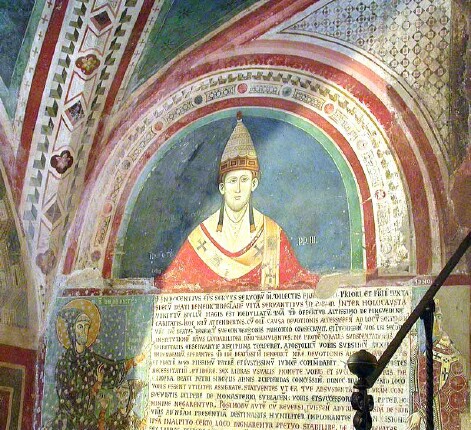The image depicts a faded fresco or wall painting, likely inside an old church, illuminated by a light source from the right. Dominating the scene is a large red and white arch. Beneath this arch stands a central figure in traditional religious vestments, wearing a conical hat and a red robe with gold draping at the top. This bearded man with brown hair, a long straight nose, and small lips looks straight ahead. Surrounding the central figure and arch are smaller, repeating L-shaped green patterns, interspersed with short segments and small cubic or circular designs, creating additional arches that layer the background.

Below the main figure, there's a substantial amount of text in black ink, written in an unfamiliar language. Flanking this text are two additional figures. On the left, a man in green clothing, possibly in a praying pose, is seen with a halo effect around his head. To the right, another figure, reminiscent of a skeleton, appears with a yellow sun-like depiction behind him. The fresco's background is a bluish hue, contributing to the aged and ethereal atmosphere of the scene. The bottom right corner of the image hints at a railing and stairs, suggesting the fresco may be situated within a larger architectural context.